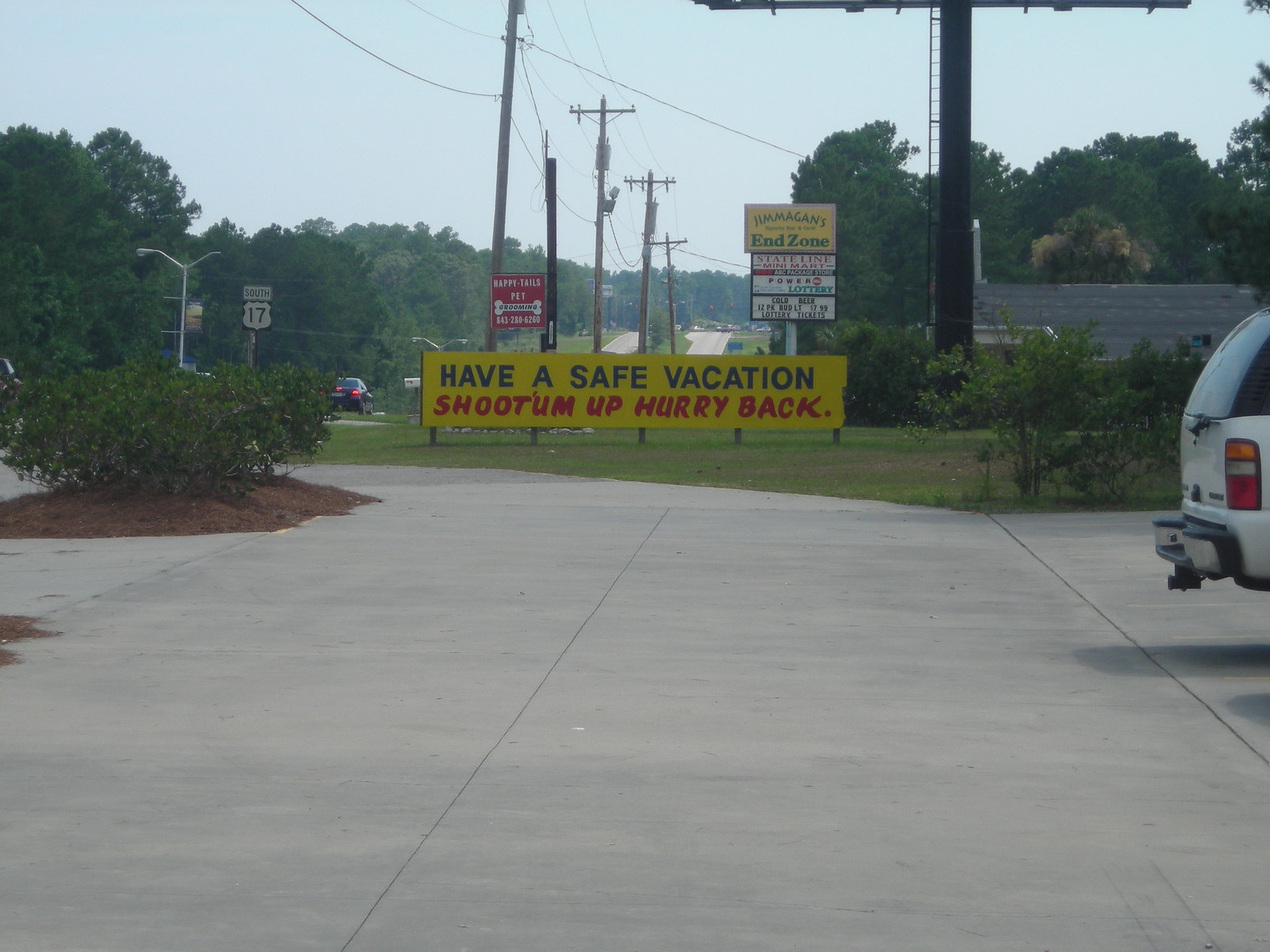In this daytime image, we are looking down a fairly long road flanked by fully grown trees with lush green leaves. Approximately 20% of the upper part of the image features a hazy grayish-blue sky. Dominating the scene is a prominent yellow billboard located in the direct middle of the lower half of the image. This billboard is relatively low to the ground and bears two messages: "Have a Safe Vacation" in blue letters at the top and "Shoot Up, Hurry Back" in red letters below. To the left of the billboard, cars can be seen driving down the road, alongside streetlights and electrical wires stretching between poles. Additional billboards are visible but their small text is unreadable. An interstate sign indicating State 17 is also present. On the right side, we notice the back of what appears to be a white Suburban parked in a driveway. The bottom middle of the image shows a large, gray cement pathway while the left middle features a dirt mound adorned with several green bushes.